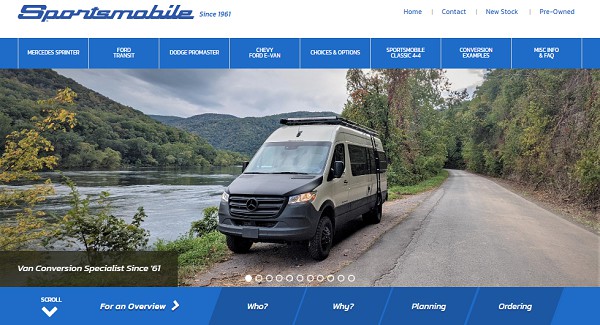Homepage of the Sportsmobile Website:

The homepage of the Sportsmobile website showcases a company rich in history, established in 1961, prominently displayed next to their name. On the top right corner, a navigation directory includes links to 'Home,' 'Contact,' 'New Stock,' and 'Pre-Owned.' 

Centrally located categories span from left to right, covering popular models and information such as 'Mercedes Sprinter,' 'Ford Transit,' 'Dodge Promaster,' 'Chevy Ford Van,' 'Choices and Options,' 'Sportsmobile Classic,' 'Conversion Examples,' 'MISC and FACTS,' among others. 

Towards the bottom of the page, additional links provide an overview of essential topics such as 'Who We Are,' 'Why Choose Us,' 'Planning Your Van,' and 'Ordering Process.' 

The main visual focus of the homepage features a high-resolution image of a Sportsmobile van. The van is parked along a road in a pristine wilderness setting, adjacent to a serene lake or river, inviting viewers to imagine adventures and the freedom of the open road. The seamless blend of detailed information and captivating imagery aims to draw users into the world of customizable, adventure-ready vehicles that Sportsmobile has perfected over the decades.